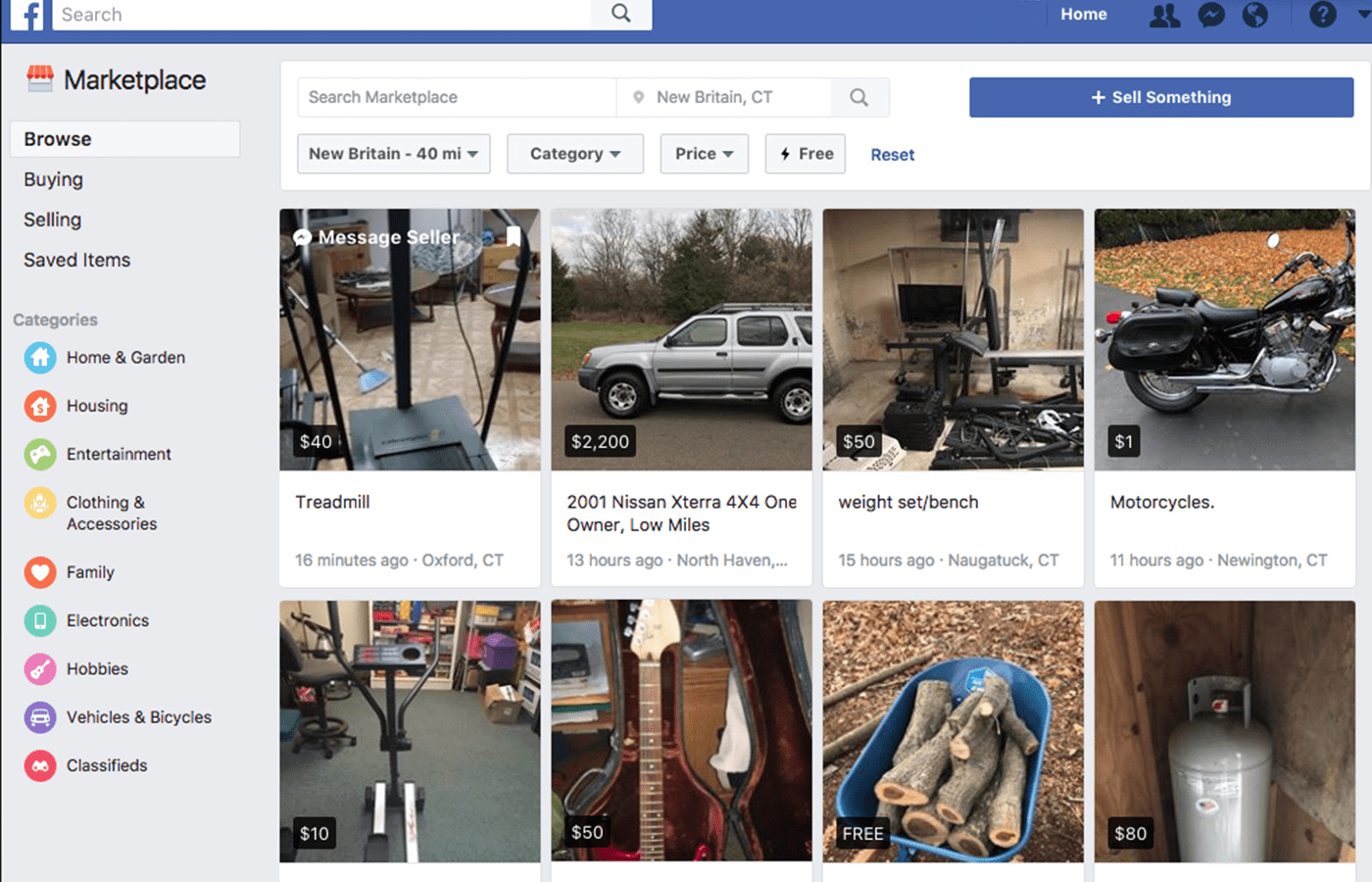The image depicts a Facebook Marketplace page displaying various items for sale. The background is predominantly white, with a gray navigation bar on the left side listing multiple categories such as Marketplace, Browse, Buying, Selling, Saved Items, Categories, Home and Garden, Housing, Entertainment, Clothing and Accessories, Family, Electronics, Hobbies, Vehicles and Bicycles, and Classifieds.

At the top of the page, the Facebook logo is prominently displayed next to a search bar. Options like "Home" and "Marketplace" are available, with "New Britain, CT" specified as the search location. A blue rectangle contains buttons for "Sell" and "Sell Something." Below this, the search radius is set to "40 miles" with filters for category, price, and a blue "Reset" button.

Eight pictures of items for sale are displayed. A highlighted item shows a $40 treadmill. Other items include a 2001 Nissan Xterra SUV listed for $2,200, described as a four-wheel-drive (4x4) vehicle with low mileage, a weight bench set for $50, motorcycles priced at $1, and a step exercise machine for $10. The "Message Seller" option is available, indicating that the user has hovered over an item.